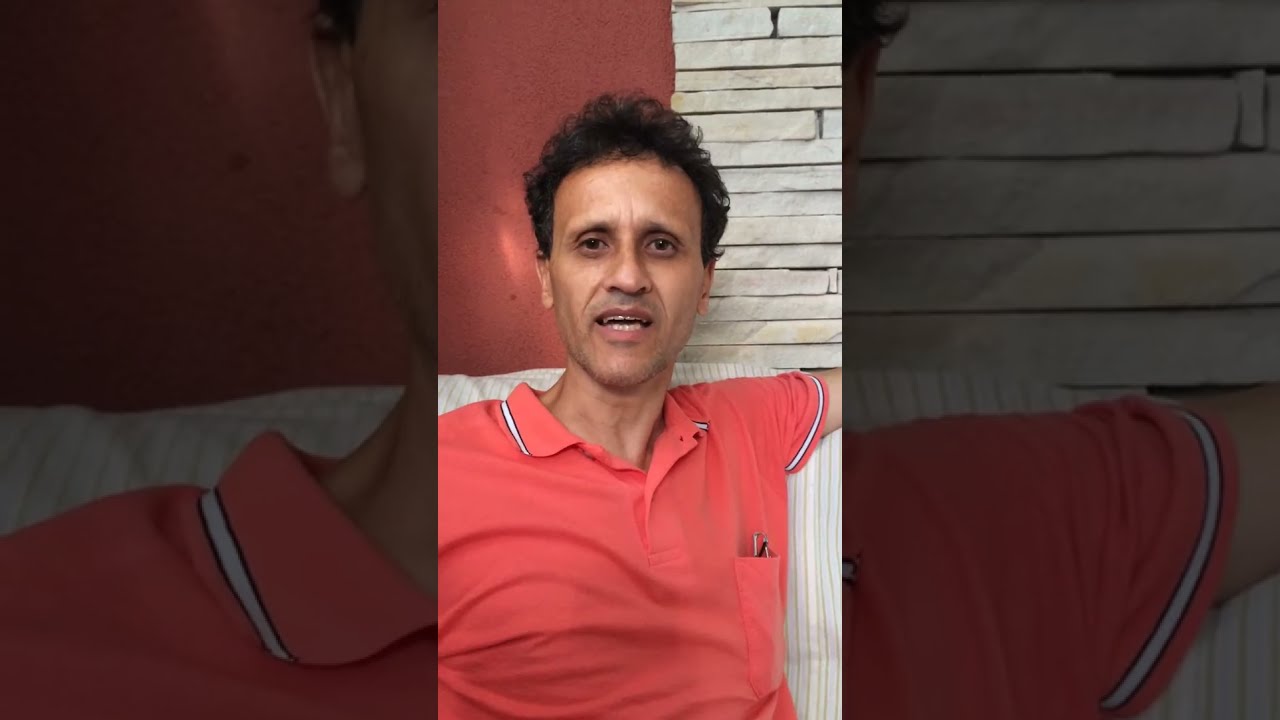The photograph, taken on a porch or patio, features a Hispanic man with a tan complexion and short curly black hair. He sports a slight 5 o'clock shadow and wears a coral pink, short-sleeve, collared shirt accented with white trim. The shirt, which has a front pocket containing a pair of glasses, stands out vividly. The man is seated on what appears to be a couch, leaning against a white pillow with thin beige stripes running vertically. He looks directly at the camera with a confused expression, his mouth slightly open. The backdrop features a distinct white wooden wall flanked by areas of red material, likely brick. The image is well-lit and of high quality, showcasing the man in clear detail, with no other people or text in the frame. The overall ambiance suggests a candid or spontaneous moment, possibly intended for social media.